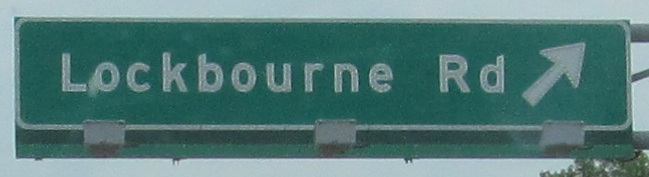This color photograph, captured outdoors in narrow landscape mode, prominently features a large green road sign with white reflective lettering and a white arrow pointing diagonally to the right. The sign reads "Lockbourne Road," with "Lockbourne" spelled out in full, L-O-C-K-B-O-U-R-N-E, and "R-D" abbreviated. The sign is bordered by a thin white line with rounded corners and is supported by a metal structure visible on the right-hand side. Three rectangular clip-like objects attach the sign to the pole. Illuminating the sign are three lights directed towards it. The background reveals a gray, overcast sky, and the top of a tree with green leaves is visible in the bottom right-hand corner.